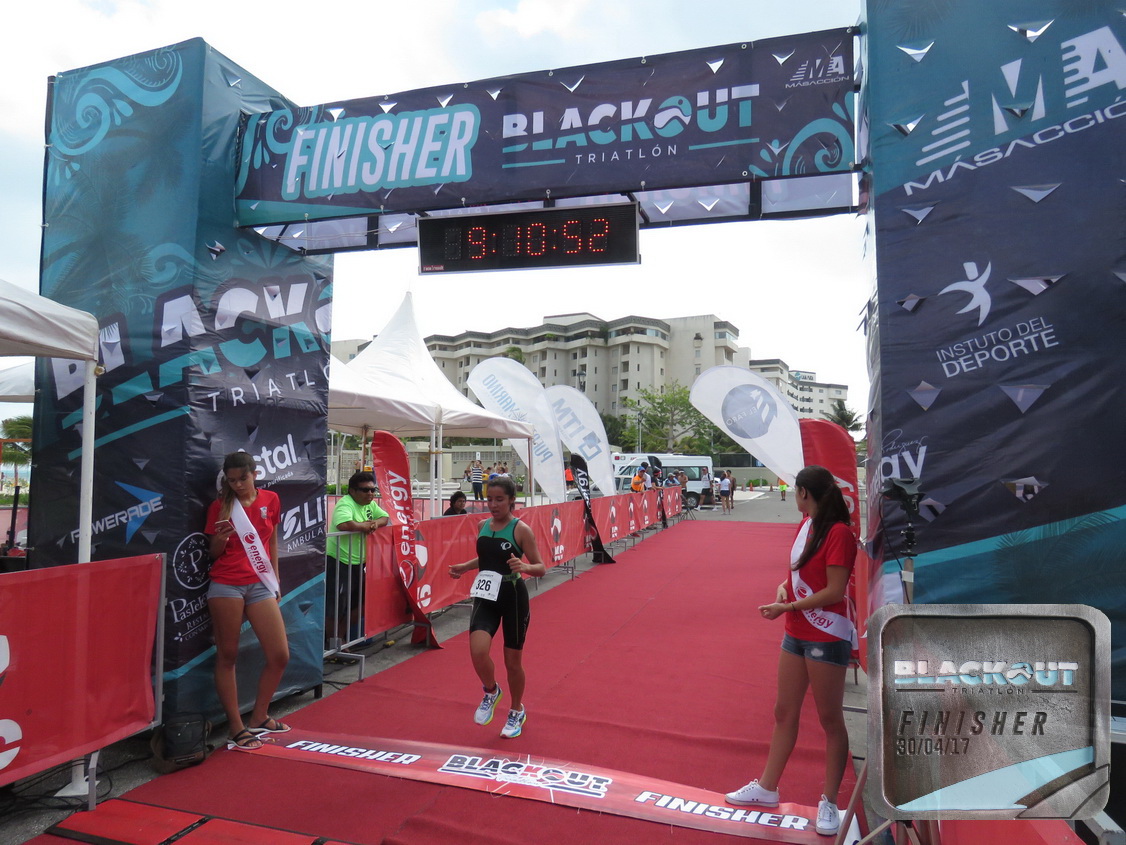This detailed color photograph captures the energetic culmination of a triathlon race at the finish line under a white sky. Dominating the scene is a blue archway adorned with light blue designs and white lettering. The archway prominently features the words "Finisher," "Blackout Triathlon," and various sponsors such as "Instituti Del Deporte" and "Black Trial," interspersed with banners. A digital clock beneath the arch shows the time "9:10:52" in orange against a black background.

A red carpet leads up to the finish line where a runner in motion, wearing a black and green outfit and a white numbered bib with "126," is at the center. To the right, two young women, likely race officials, are wearing red shirts, blue shorts, and white sashes. One appears engrossed in her cell phone. Beyond them, a man in a yellow-green shirt can be seen. The background showcases gray buildings, possibly a hotel, and a white tent alongside fencing covered with banners, delineating the race area. This vibrant and dynamic moment encapsulates the triumphant end of a race against the backdrop of urban structures.